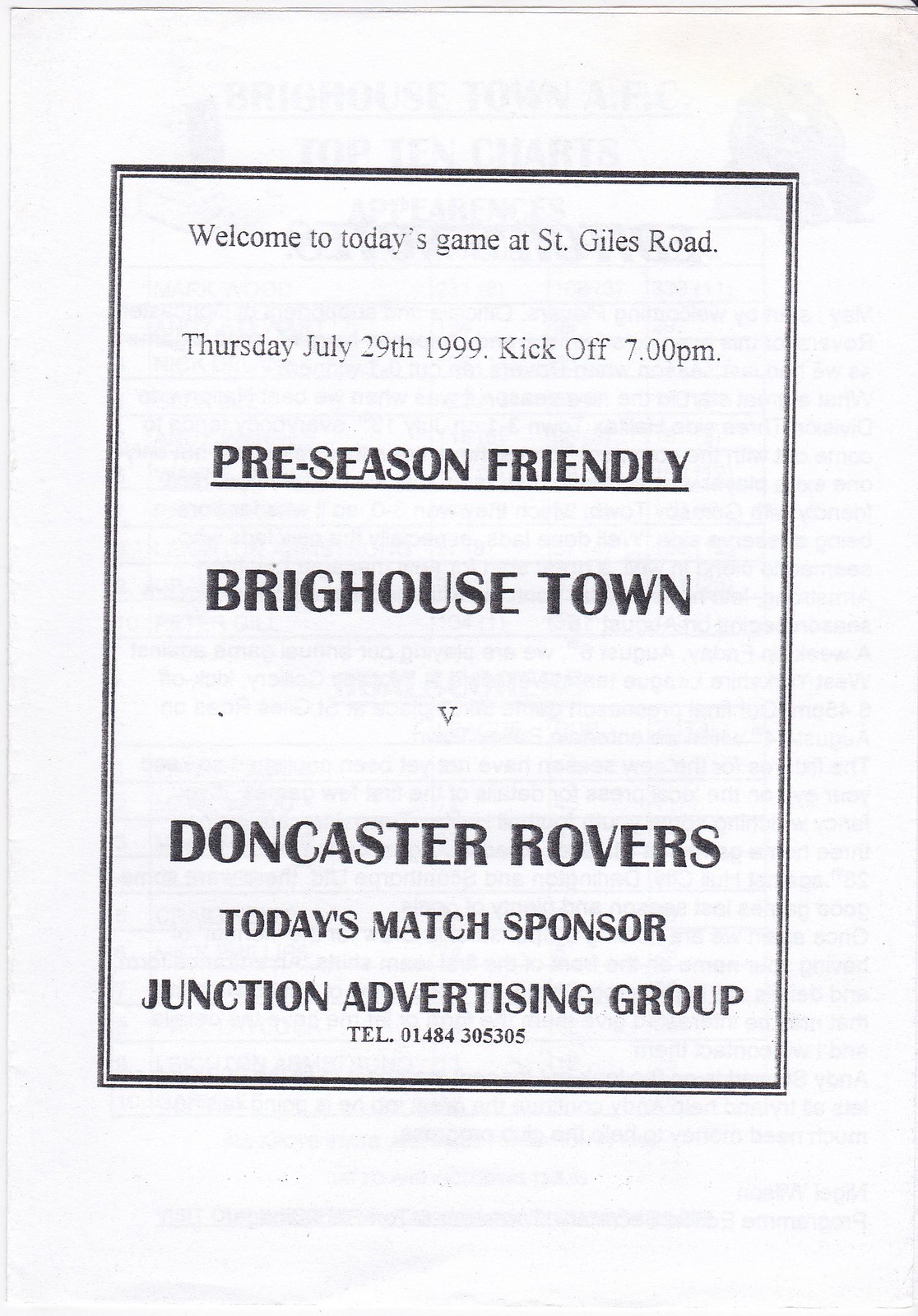The image depicts a vintage poster framed with a light black border, announcing a soccer match predominantly in gray to black lettering on a white background. At the top, it reads "Welcome to today's game at St. Giles Road." Below that, the date and time are listed as "Thursday, July 29th, 1999, kickoff 7.00 p.m." In larger black letters, the poster highlights "Pre-Season Friendly" with a black line beneath. Following that, the teams "Brighouse Town" and "Doncaster Rovers" are noted, separated by a light "V" symbol. Toward the bottom, it mentions "Today's Match Sponsor: Junction Advertising Group," followed by their telephone number, "TEL: 01484 205 305."